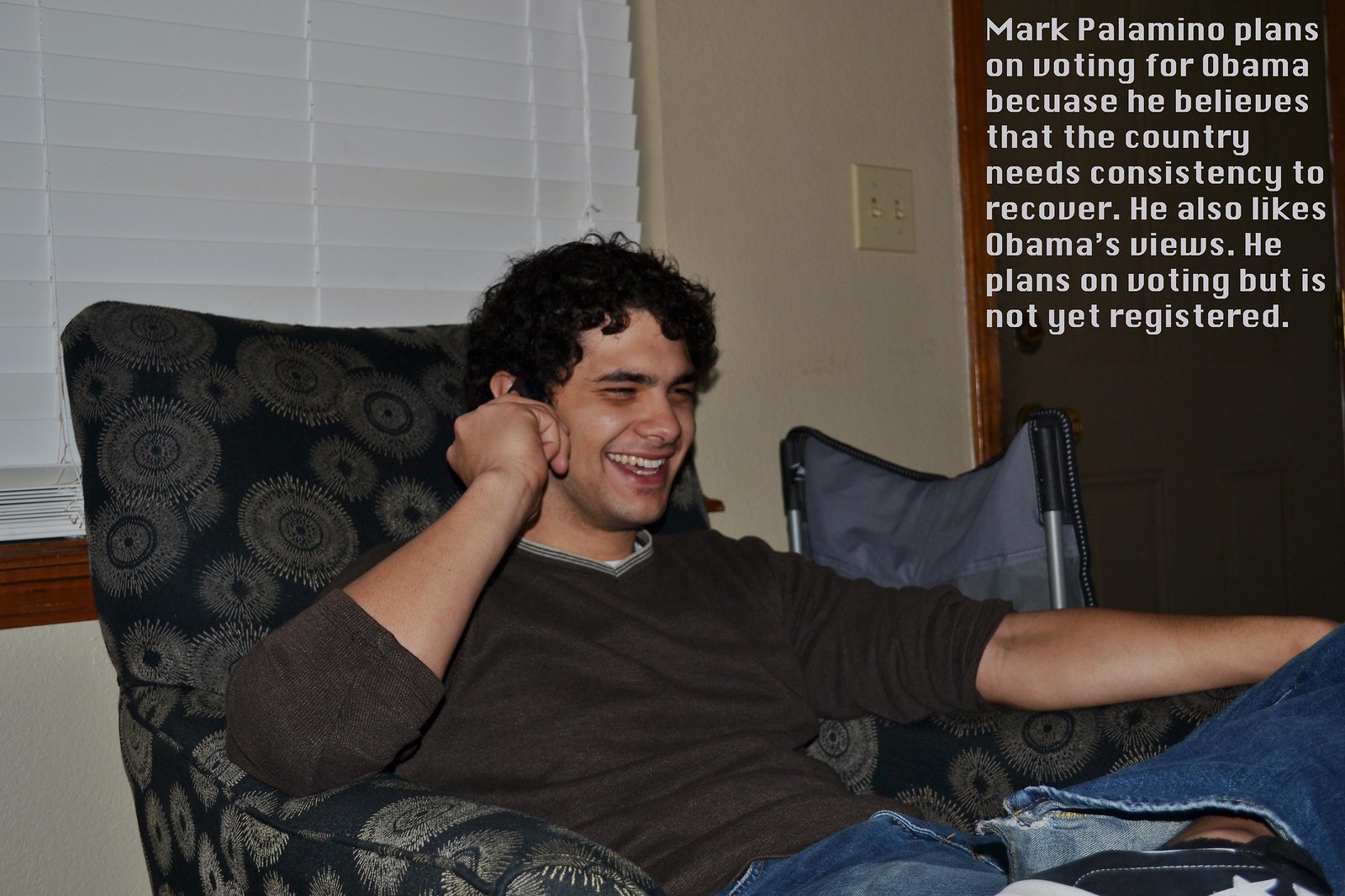In this photo, taken indoors—likely in a living room—we see a young man sitting comfortably in a chair with a distinct black-and-white pattern that resembles fireworks. The chair is positioned in front of a window with white blinds. Adjacent to him is a fold-out chair resembling those often taken to the beach. The man, Mark Palamino, has dark curly hair and is wearing a dark gray (or possibly brown) long-sleeve shirt with the sleeves rolled up, paired with blue jeans. He is depicted in a relaxed pose with one leg crossed over the other, and his eyes are partially closed as he laughs. His footwear features a design with white stars. The top right corner of the image contains white text that reads: "Mark Palamino plans on voting for Obama because he believes that the country needs consistency to recover. He also likes Obama's views. He plans on voting but is not yet registered." This caption suggests efforts to promote voter registration and support for Obama, likely contextualized around the 2008 election.